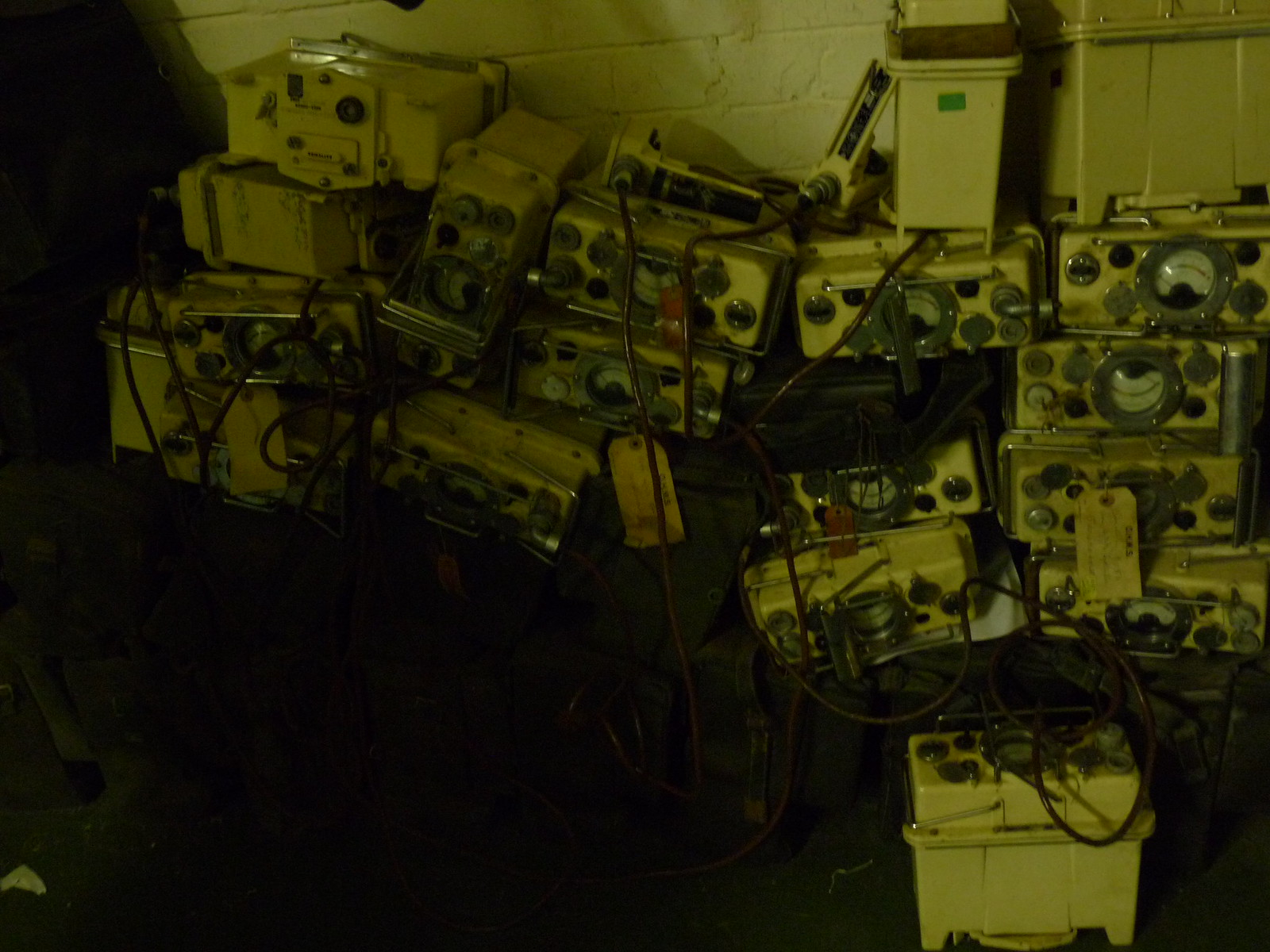The photograph depicts a dimly lit room, possibly a basement, with a white-painted cinder block wall serving as the backdrop. The floor is cluttered with several piles of old-fashioned radio or electronic equipment, which are largely beige with brushed silver central panels. Each piece features a prominent round metal dial, adorned with black and silver knobs, and displays a gauge or graph that likely measures some parameter such as speed or power. Antennas and handles protrude from the tops of the rectangular devices. In total, there are around five piles, each stacked four or five units high, with cables draped over some of them. One piece of equipment, bathed in a faint yellowish light, is positioned separately in a darkened part of the room, adding to the overall sense of disarray.